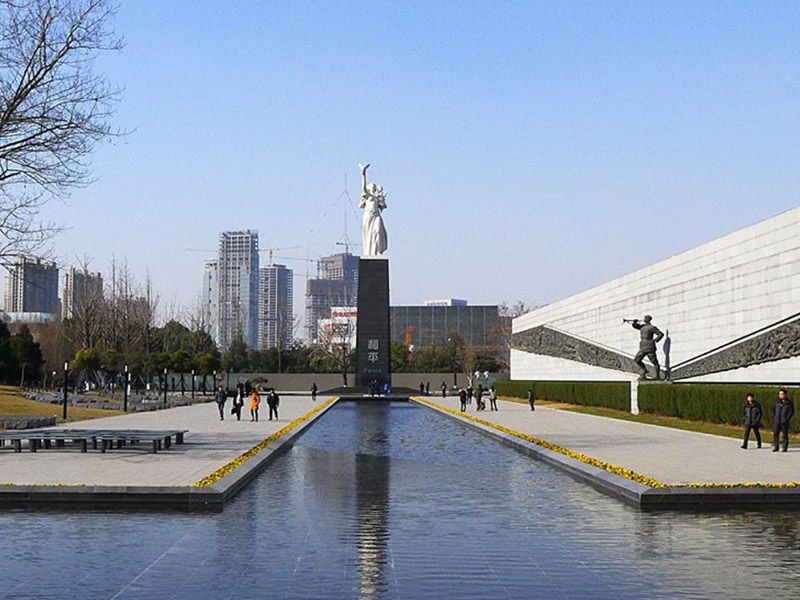The photograph depicts a public monument resembling the Washington Monument, situated in a historical area bustling with visitors. The focal point is a tall, black obelisk topped with a statue of a woman in a flowing dress, holding what appears to be a dove. This monument stands at the center of a shallow pool, flanked by paved concrete walkways and benches. To the right, there's a white wall adorned with a statue of a soldier holding a trumpet or bugle. The background reveals several city skyscrapers, many still under construction, adding an urban contrast to the historical ambience. Amidst the lively scene, visitors can be seen strolling and taking pictures, highlighting the location's appeal as a tourist destination.